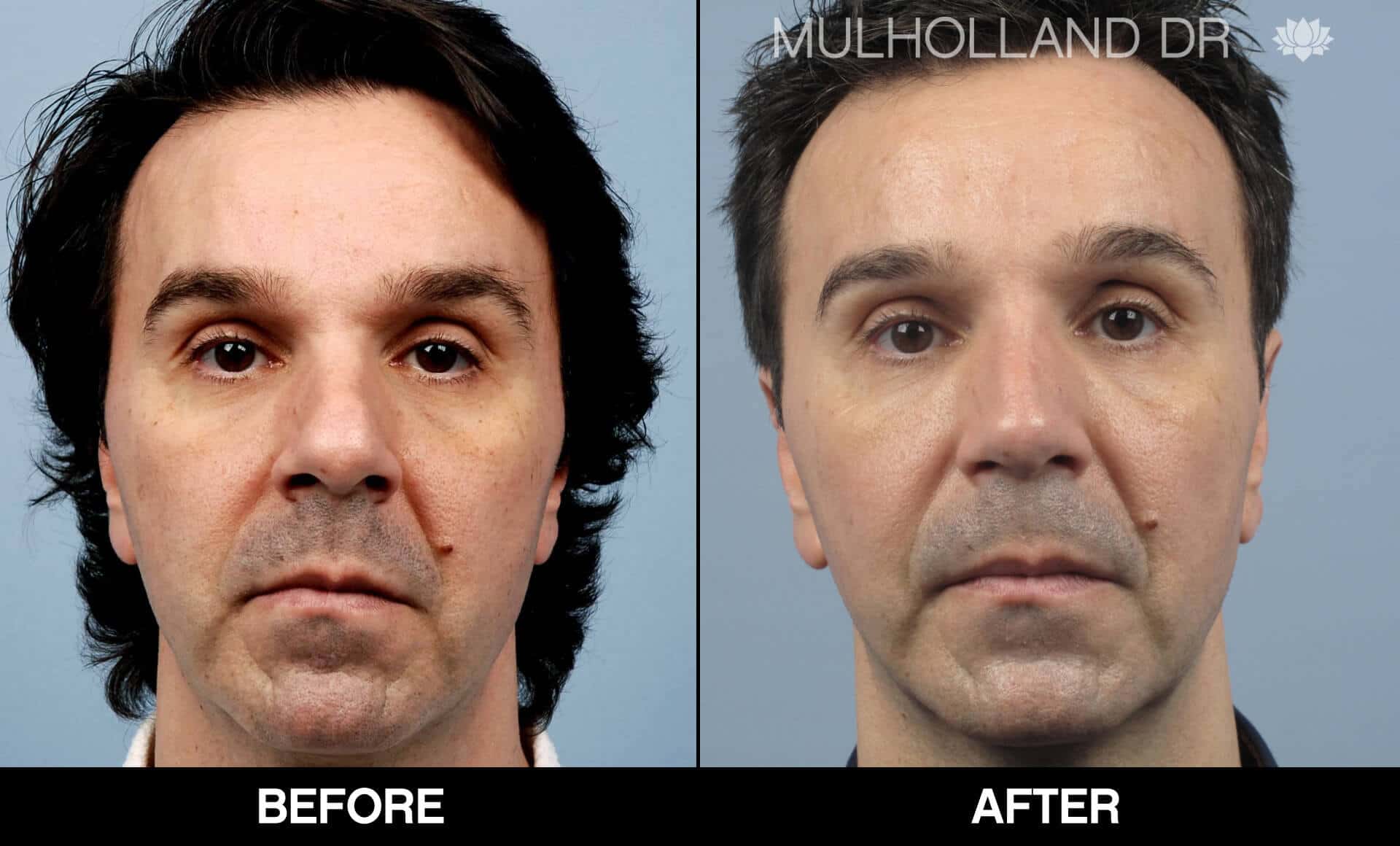The photograph depicts a before-and-after transformation of the same middle-aged, white man with changes in his appearance suggesting cosmetic enhancements. At the top of the image, the text "Mulholland Drive" is prominently displayed, while a black bar at the bottom labels the photos "before" and "after." 

In the "before" picture, positioned on the left, the man sports longer, dark hair reaching down to his collar. His complexion appears ruddy, and he seems slightly heavier with a tired expression. This image also features harsher lighting, highlighting his more pronounced wrinkles and the width of his nose.

Conversely, the "after" photo on the right shows the same man with shorter, lighter hair and a more refined appearance. His skin looks healthier, possibly due to cosmetic procedures such as a nose job and wrinkle fillers, giving him a thinner and refreshed look. The lighting in this image is softer and slightly blurred, further enhancing the improvements in his appearance. 

Overall, the transformation is meticulous, highlighting significant enhancements in the man’s facial features and overall demeanor.